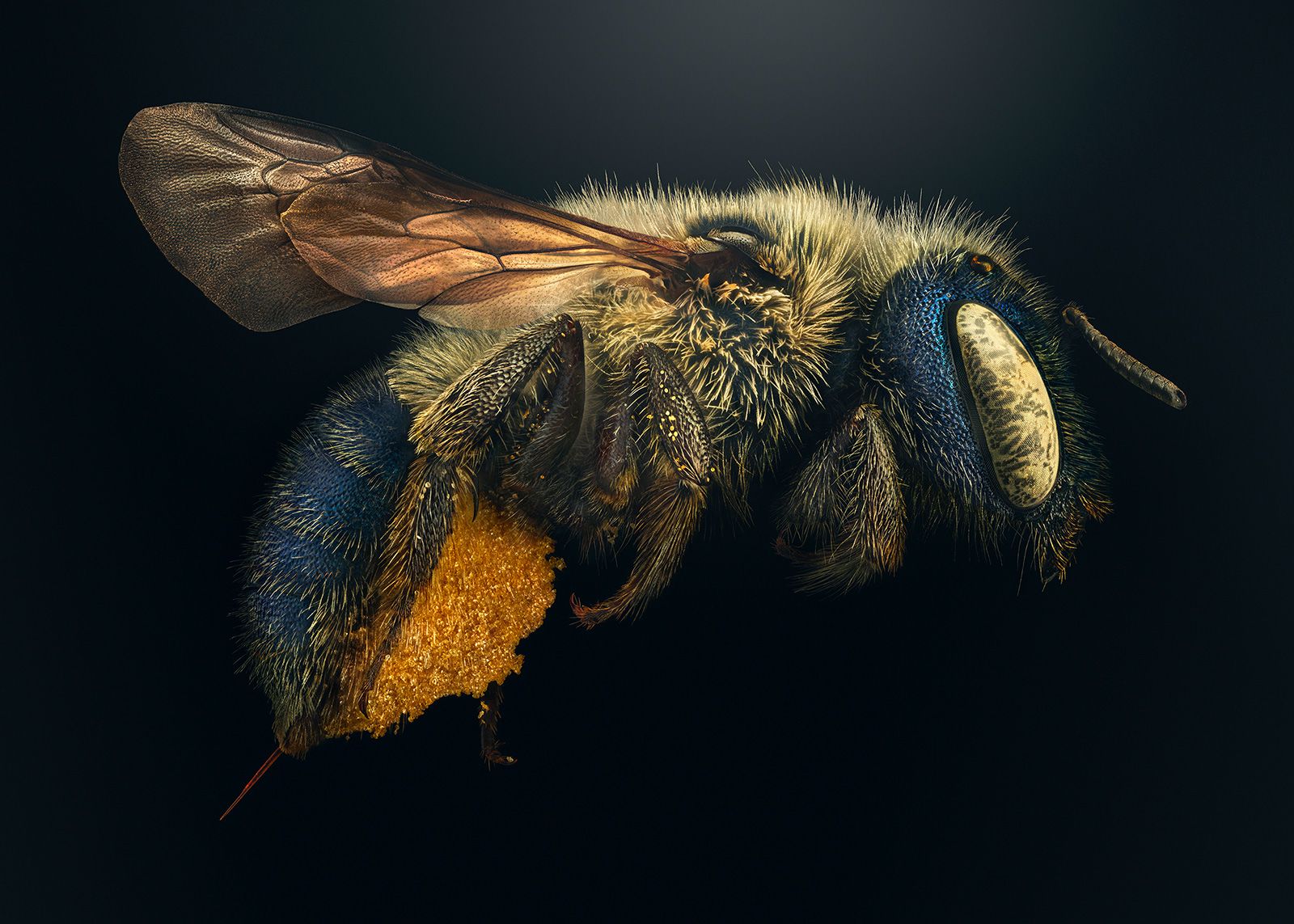The image depicts a highly detailed, almost lifelike close-up of an insect against a stark black background. The creature, which might be a honeybee or possibly a type of fly or hornet, is displayed in vivid color with intricate features that give it an almost holographic or digitally generated appearance. The insect’s body is covered with short, spiky yellow and blue fuzz, adding to its furry look. Its oblong, tannish eyes are accented with zigzags of gray-black and a blue outline, while its wings are translucent with a coppery hue, showing no signs of movement as they are tucked back. The insect's underside is bright yellow, and its back tail is blue with protruding yellow tips that could be mistaken for pollen. It also has a distinctive, sharp stinger at its rear end. The legs are curled under its lifeless body, suggesting that the insect is dead. The overall magnified and color-enhanced effect of the image contributes to its surreal quality, capturing the viewer's attention with its lifelike yet otherworldly presentation.